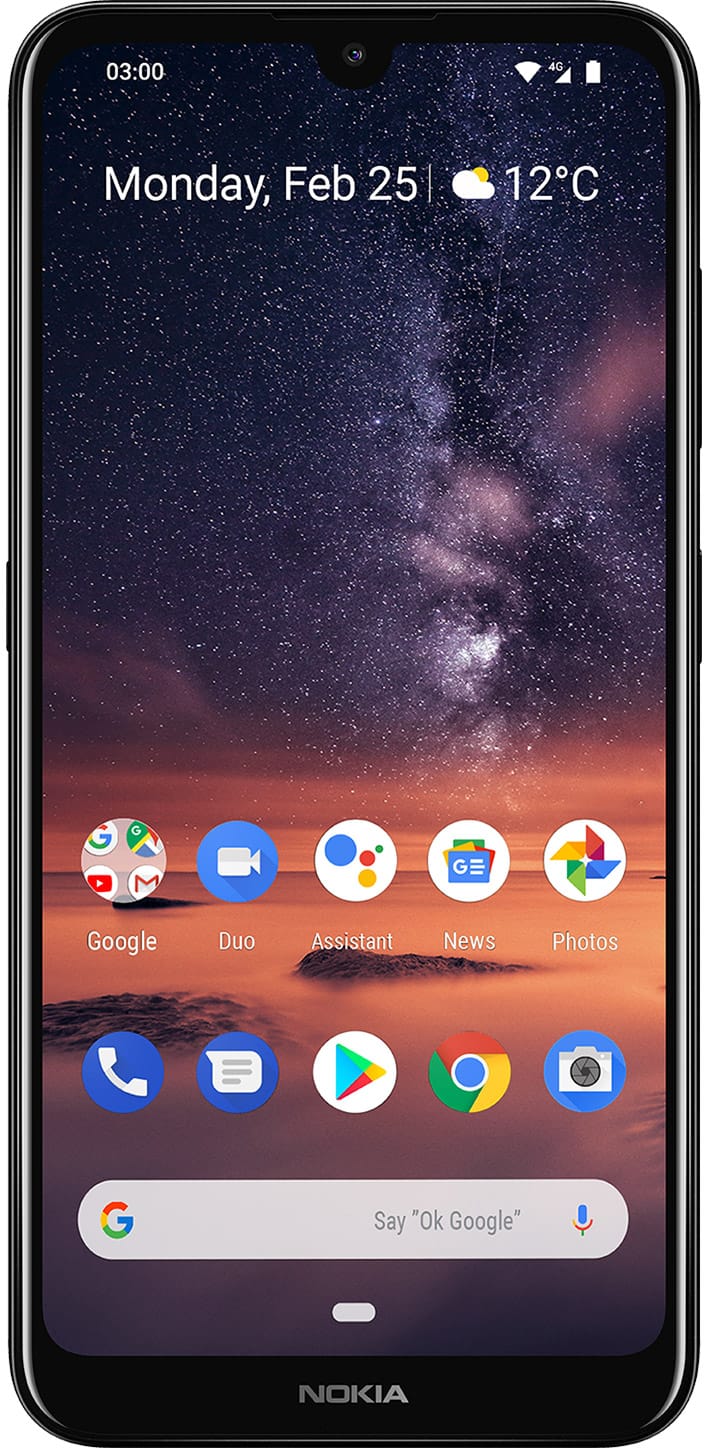**Detailed Caption:**

The image showcases a smartphone screen against a completely white background, resembling a product image meant to highlight the display features. The screen displays the time in military format as 03:00, indicating it is 3 a.m. The status bar at the top right shows that the phone is fully charged, with the battery icon filled in white. The date is prominently displayed as Monday, February 25th. Additionally, a small weather widget reports partly sunny or mostly cloudy conditions with a temperature of 12 degrees Celsius.

The smartphone's background is a stunning, space-themed composition. The lower part of the wallpaper features a serene sunset over an ocean, transitioning into a clear night sky adorned with numerous stars and wispy, galaxy-like clouds.

On the home screen, several apps are docked at the bottom: a Google app, a video camera app, and a photo gallery app, hinting at the phone's multimedia capabilities. This detailed representation captures the essential information one would see on the display of this smartphone model.